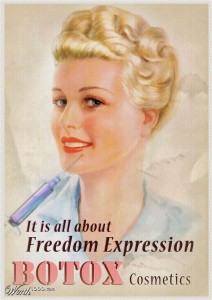The magazine cover features a detailed advertisement for Botox, centered around a 1920-1940s style woman with short, tightly curled blonde hair that doesn't extend past her ears. Her hair is pressed closely to her head, giving a classic vintage look. She has light pale skin and prominent red lips, flashing a smile that reveals her top teeth. Her eyes are directed towards the viewer, and she has thin brown eyebrows. She is donning a baby blue shirt that heightens the nostalgic aesthetic.

A blue needle is prominently depicted, pointing at her face and piercing the area just below her lower lip but above her chin, symbolizing the Botox procedure. The background of the cover is primarily beige with a thin light gray border encasing the image, adding to the minimalist and elegant design.

Text on the cover is as follows:
- "It's all about freedom expression" in black text, indicating the self-expressive nature of cosmetic enhancements.
- "Botox" in large pink font, drawing attention to the primary focus of the advertisement.
- "Cosmetics" in a smaller black font beneath it, tying the whole theme together.

The overall composition of the magazine cover creates a striking blend of vintage charm and modern cosmetic advertising.